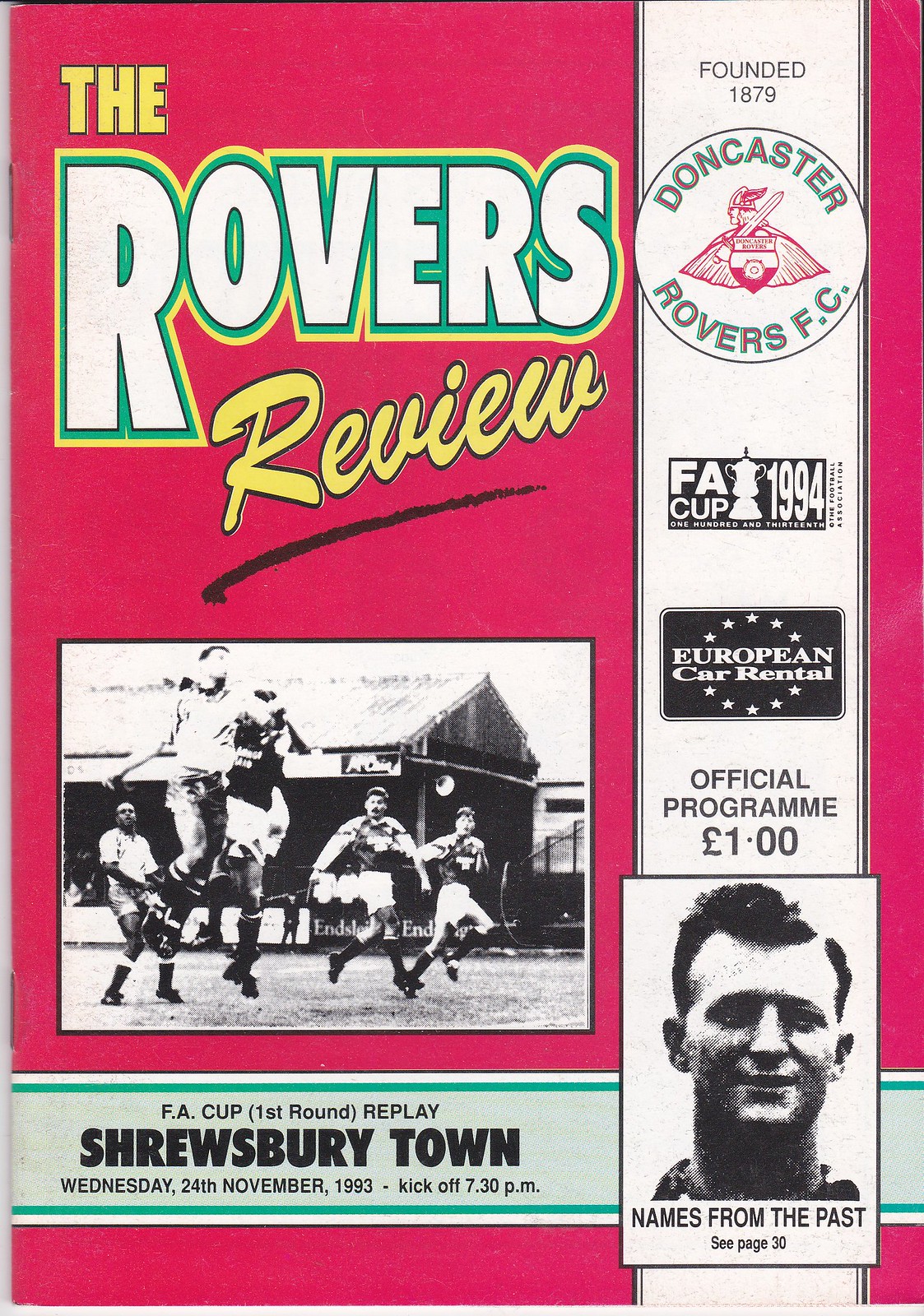This magazine cover appears to be a classical "Rovers Review," an official program from the Doncaster Rovers Football Club, founded in 1879. The cover features a distinctive pinkish-red background with a white vertical banner running along the right edge from top to bottom, emblazoned with "FOUNDED 1879" and multiple logos, including the club's emblem. 

In the top left corner, the word "THE" is prominently displayed in large yellow capital letters. Below it, "ROVERS" is written in white letters outlined in green and yellow. Underneath "ROVERS," the word "REVIEW" is diagonally positioned in yellow and underlined with a black mark. Centrally placed is a black-and-white photograph of players on the field, overlaid with a horizontal green banner that states "F.A.C. (FIRST ROUND) REPLAY." Below this, "SHREWSBURY TOWN" is boldly printed in large black capital letters, with smaller text beneath it detailing the match date, "WEDNESDAY, 24TH NOVEMBER, 1993," and the kickoff time, "7:30 PM." 

Additionally, the cover advertises the program’s price as "OFFICIAL PROGRAM £1.00," and another black-and-white photograph of a young man is present below the main image. The background description mentions the team logo featuring prominently in red and a note highlighting sponsors of the day. All photographs display scenes of players on the field, enhancing the program's nostalgic and historical value.